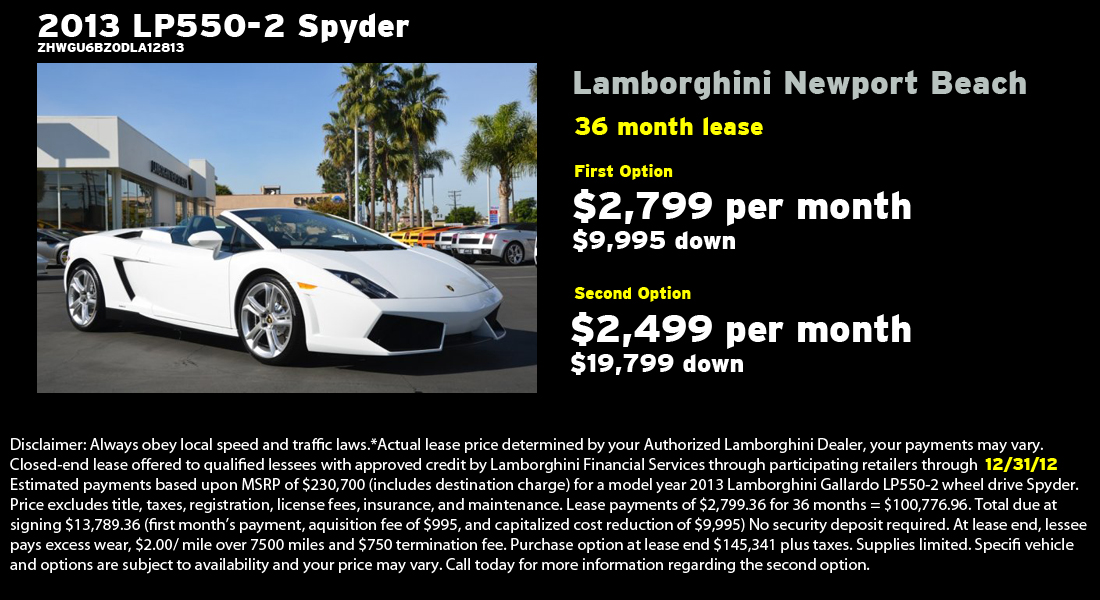The image is a car advertisement set against a black background, featuring prominent white and yellow text. Dominating the upper left quadrant is a color photo of a sleek white convertible, potentially a Lamborghini, parked at an auto dealership lot amidst palm trees and other cars. The car, angled slightly to the right, is specifically identified at the top in white text as a "2013 LP 550-2 Spyder," followed by a serial number "ZH WGU 6BZ ODL A12813." To the right of the photo, additional text highlights the offer details: "Lamborghini Newport Beach, 36 month lease" in grey, yellow, and white text. Two leasing options are provided: the first at $2,799 per month with $9,995 down, and the second at $2,499 per month with $19,799 down. Some legal disclaimers in small white text at the bottom mention adhering to speed and traffic laws, and encourage contacting for more details regarding the second option.